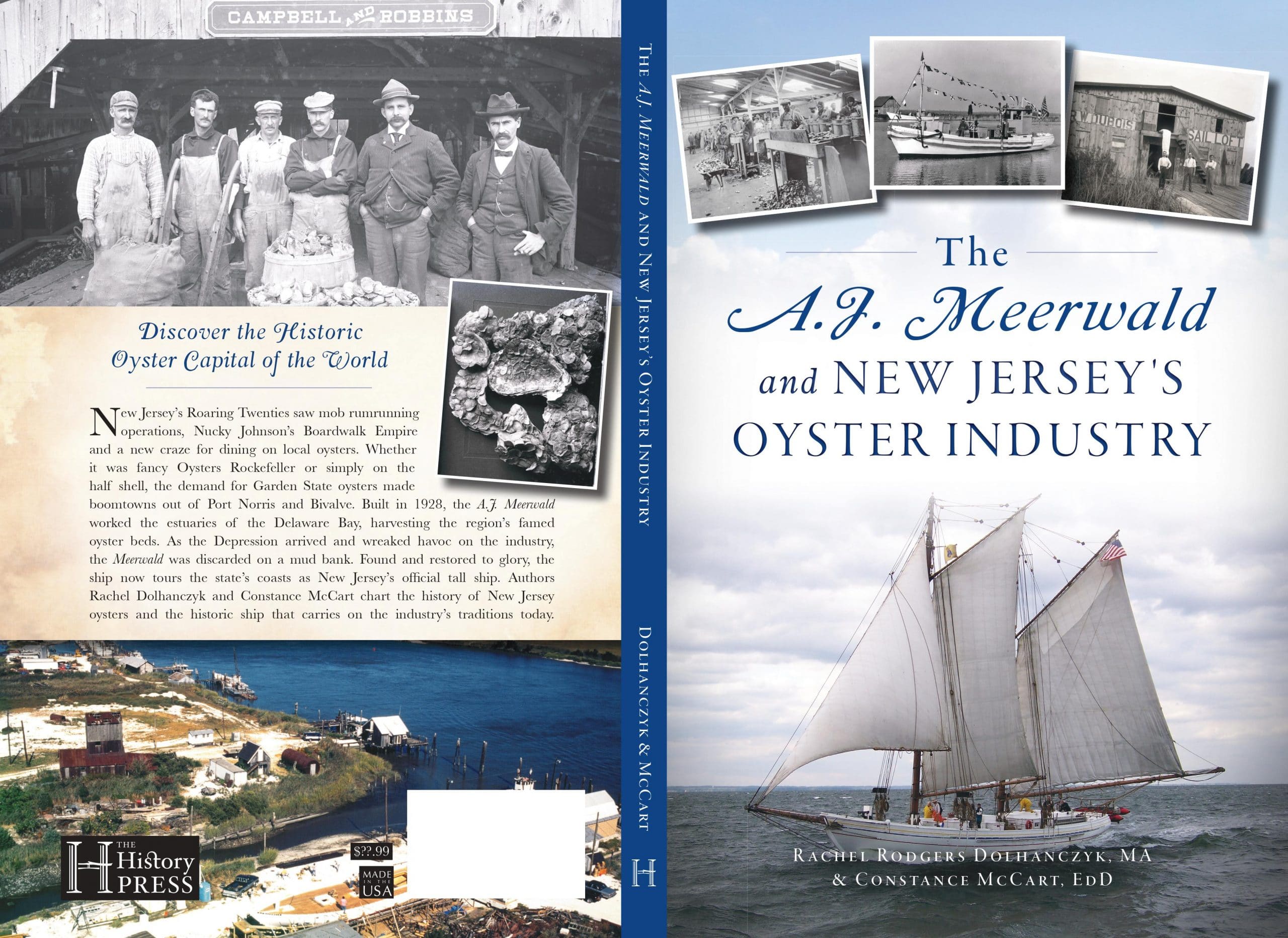This detailed poster or book cover features a vibrant collage of images and text, providing a rich historical insight into New Jersey's oyster industry. On the left side, the cover showcases a black-and-white photograph of six people standing around piles of oysters. Beneath this image, a paragraph with the heading "Discover the Historic Oyster Capital of the World" details New Jersey's Roaring Twenties, including mob-run rum operations, Nucky Johnson's Boardwalk Empire, and the novel allure of dining on local oysters, whether as Oysters Rockefeller or simply on the half-shell. This text underscores how the demand for Garden State oysters transformed towns like Port Norris and Bivalve into boomtowns.

Below this paragraph, there is an aerial photograph of a town with a prominent water board visible. At the bottom left corner, 'The History Press' is printed. Moving to the right side, the top displays three black-and-white photographs: the exterior and interior of a factory and a boat. Text in blue beneath these images reads, "The A.J. Meerwald and New Jersey's Oyster Industry." The background image across the right side is a sailing boat navigating the sea. Notably, the names Rachel Rogers, Dolhan Czech, M.A., and Constance McCart, E.D.D., are printed prominently, indicating the authors who chart the history of the A.J. Meerwald and the oyster industry.

A blue vertical strip runs between the left and right sides of the cover, adorned with vertical text reading, "The A.J. Meerwald and New Jersey's Oyster Industry, Rachel Rogers, Donna Chatz, M.A., and Constance McCart, E.D.D." The narrative details the A.J. Meerwald's construction in 1928, its role in harvesting Delaware Bay's famous oyster beds, and its eventual restoration after being sidelined by the Great Depression. Now, New Jersey's official tall ship, the A.J. Meerwald continues to honor the state’s oyster industry legacy.